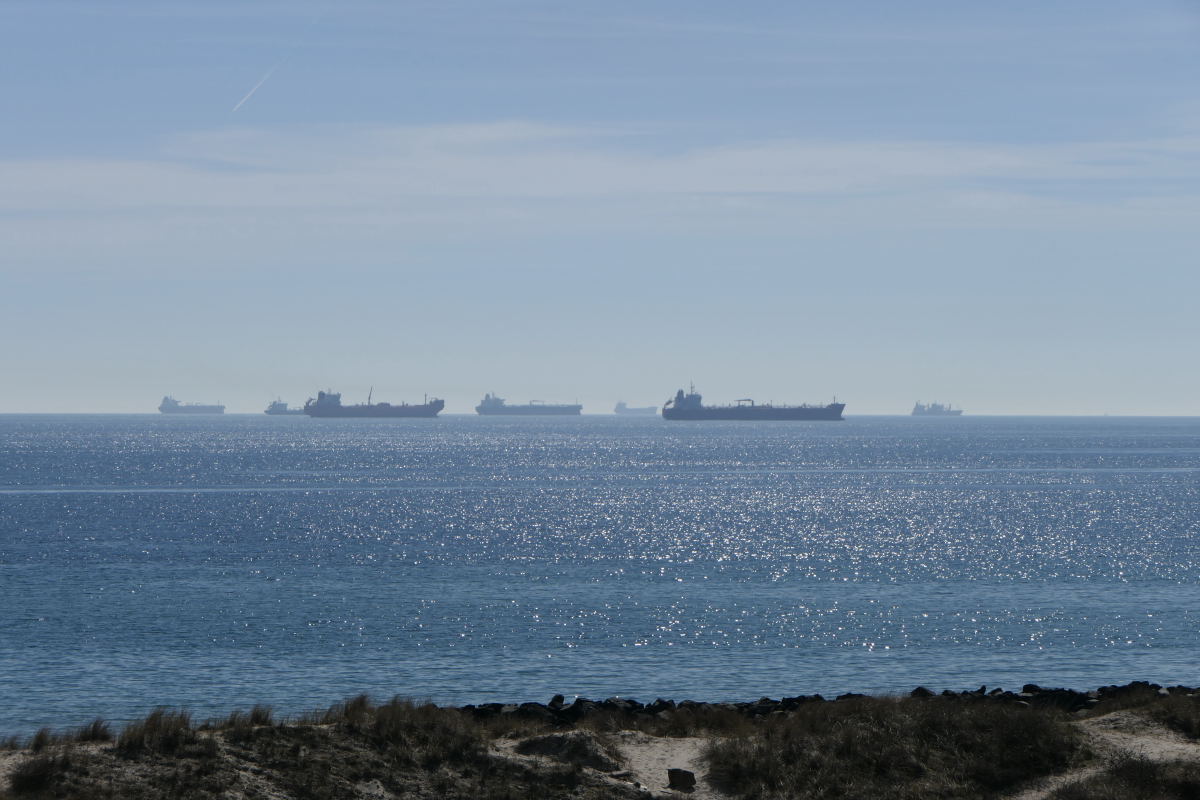This outdoor image captures a serene oceanic scene beneath a medium to light blue sky interspersed with soft white clouds. The calm, deep blue ocean stretches out towards the horizon, where sunlight reflects off the water, creating shimmering highlights. Distant on the skyline are seven large boats, likely barges, all directed towards the right. They vary in size, with the closest being larger and those further away appearing smaller and partially obscured by haze. The foreground features a strip of sandy land adorned with patches of greenery, suggesting the vantage point is slightly elevated, providing a downward perspective on the tranquil maritime vista.